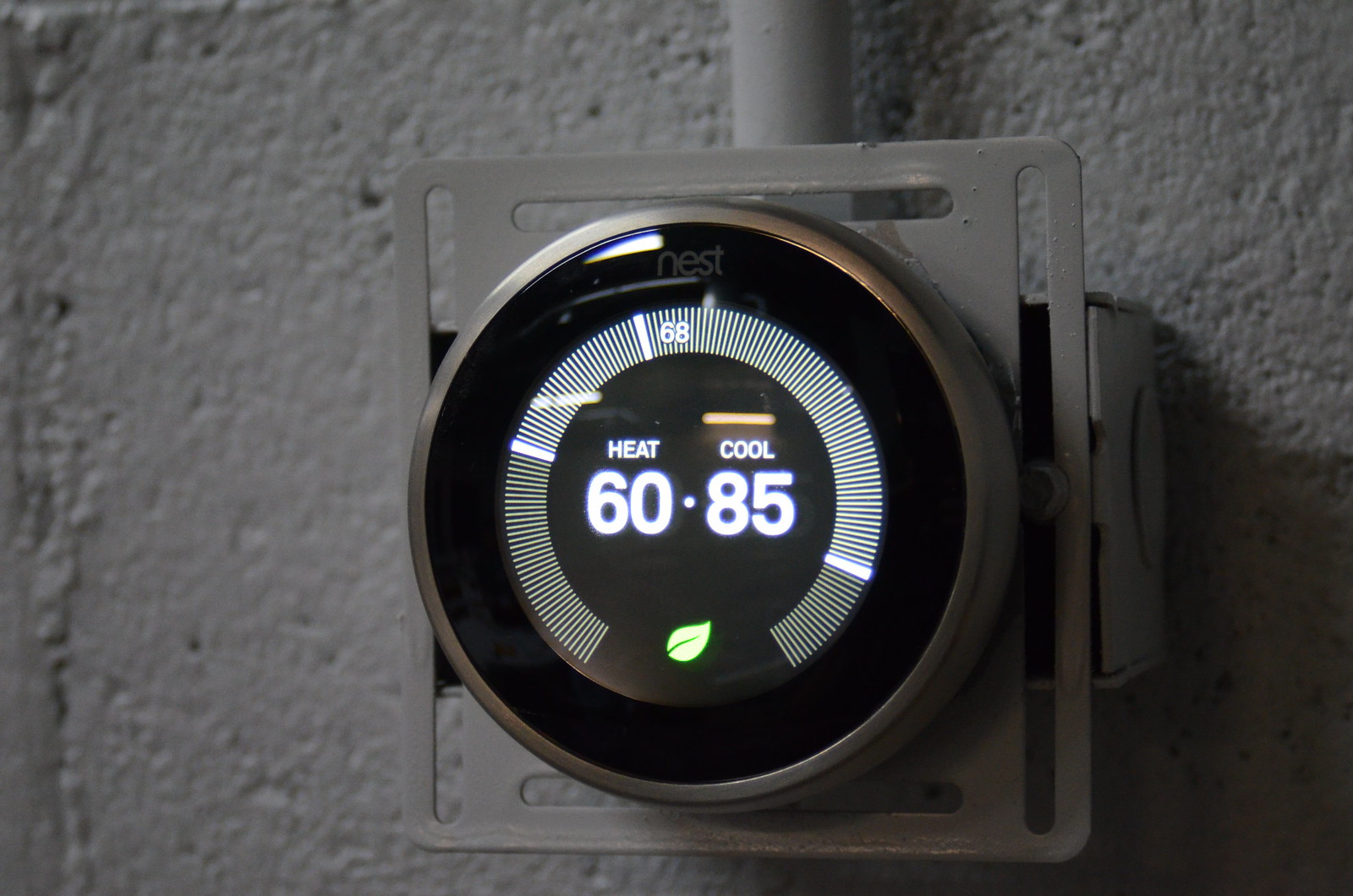The image features a digital thermostat, prominently identified as a Nest thermostat, designed for heating and cooling. This device is affixed to a gray-painted cinder block wall. Extending from the top of the thermostat is a conduit for electrical wiring, leading to a square metal box situated directly above the device.

The thermostat itself is characterized by a large, round knob with a silver outer ring. The center of the thermostat displays the brand name "Nest" at the top, enclosed within a black circular face. Encircling the outer edge of the face are numerous individual white lines, forming a virtually complete circle save for a small gap at the bottom. Within this gap, a green leaf icon is illuminated, signifying energy efficiency.

In the very center of the display, white-lit letters indicate "heat" and "cool." Directly below "heat," the number "60" is prominently displayed, followed by a dot, while beneath "cool," the number "85" appears in equally large numbers. An additional yellow line is visible above the "cool" setting. The thermostat also reflects some ambient light, adding to its sleek appearance.

Positioned slightly off-center toward the top of the circular display, one of the white lines is illuminated, with the number "68" glowing in the middle, indicating the current temperature setting.